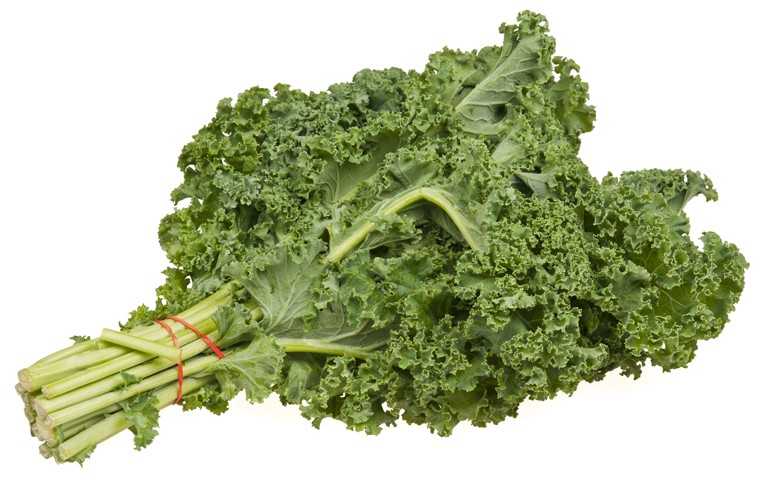A detailed image depicts a bunch of dark green leafy vegetables, most likely mustard greens, bound together by two medium red rubber bands. The vibrant green leaves form a broad, dense canopy at the top, while the light green stalks, resembling celery in color, point roughly to the two o’clock position. The stalks are uniform in length, with a total of around 15 to 20 bundled together. One of the stalks appears broken and leans to the side. The leaves, though healthy, appear slightly wilted, with their ruffled edges bending forward. The underside of the leaves is slightly dustier than the front. The composition rests against a clean white background, highlighting the details of the vegetable bundle.